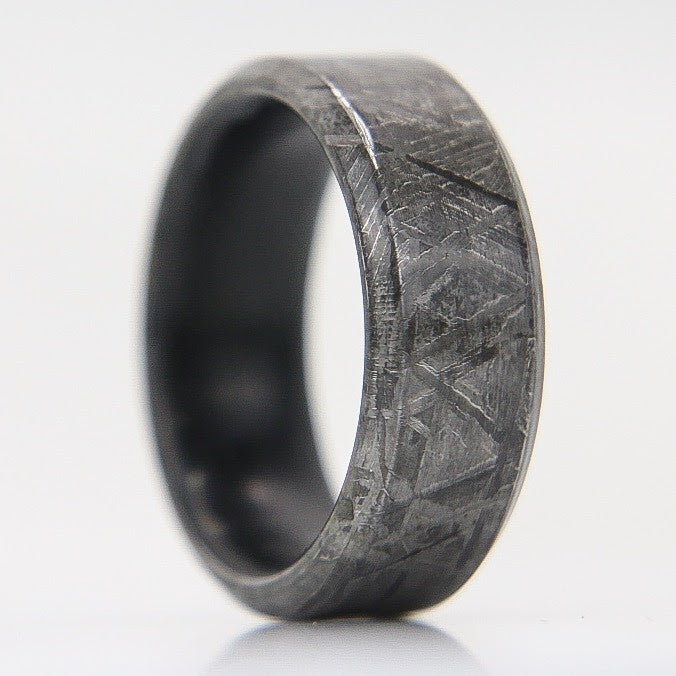In this detailed image of what resembles a standing tire, we see a prominently featured ring that occupies the majority of the frame. The background of the image is a stark white, enhancing the focus on the ring itself. The ring, primarily platinum gray in color, has a substantial thickness of about an inch and a half. Intricate carvings and a diagonal design adorn its surface, giving it a textured appearance. Notably, the inner part of the ring is a darker gray. The ring is positioned upright, casting a distinct shadow below it, and there is a visible area at its top that appears to have been damaged or hit, adding an element of wear.